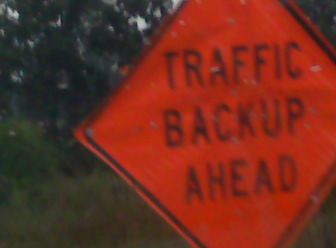The image captures an outdoor scene with a somewhat indistinct background that could possibly be a dense hedge or a tree line. The bottom portion of the photograph shows lighter green hues, suggestive of a grassy area. Dominating the majority of the frame, there's a prominent, diamond-shaped traffic sign, oriented on one of its points. The sign itself is a striking red color with bold black lettering, clearly designed to grab the attention of motorists. The message on the sign appears to caution drivers, suggesting their best course of action would be to turn around. The scene is faintly illuminated, creating a stark contrast between the lush green grass and the dark foliage in the background.